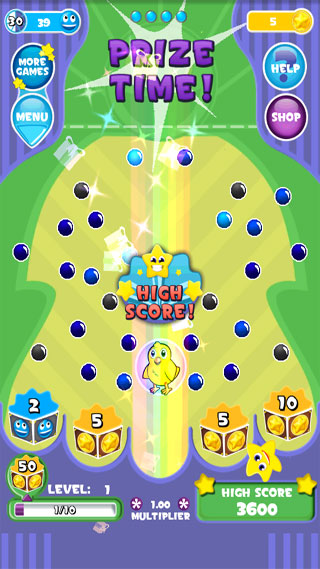The image appears to be a screenshot from a mobile game, potentially resembling a pinball-style game, though its exact nature remains unclear without playing it. The screenshot is in portrait orientation, suggesting it was taken on a phone.

At the top of the image, in purple text, there’s the phrase “Prize Time!” with an exclamation point. In the upper left corner, there is a button labeled “More Games” followed by “Menu.” In the upper right corner, there are buttons marked “Help” and “Shop.”

Just below these icons, towards the bottom, the game displays “Level: 1” along with a status bar indicating the player's progression. To the right of the status bar, the high score is prominently shown as "High Score: 3600."

Overall, the layout of buttons and text suggests an engaging and interactive game interface, organized neatly for easy navigation and play.